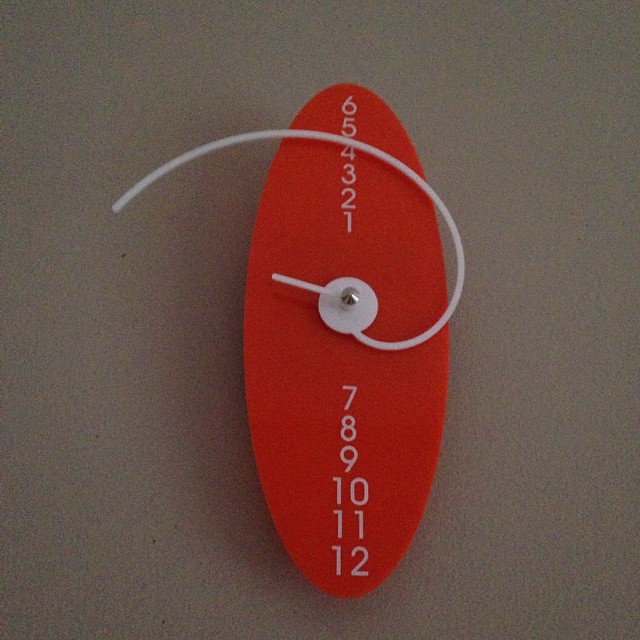The image features a distinctive and intricate clock design. On the left side, there is a gray ball that appears to represent the hour hand. Adjacent to it, a surfboard-like element is present, with numbers arranged sequentially on both the top and bottom halves—1 through 6 on the top and 7 through 12 on the bottom. Centrally located, a silver pin holds a circular piece from which a line extends. This line twists and turns, eventually forming a large white circle that encompasses the entire design in a curvaceous stripe. The clock's unconventional mechanism features a long wire that changes its position, seemingly indicating the hours in a fluid and dynamic manner. The unique aspect of this clock is that it solely displays the hour hand in a creative configuration.